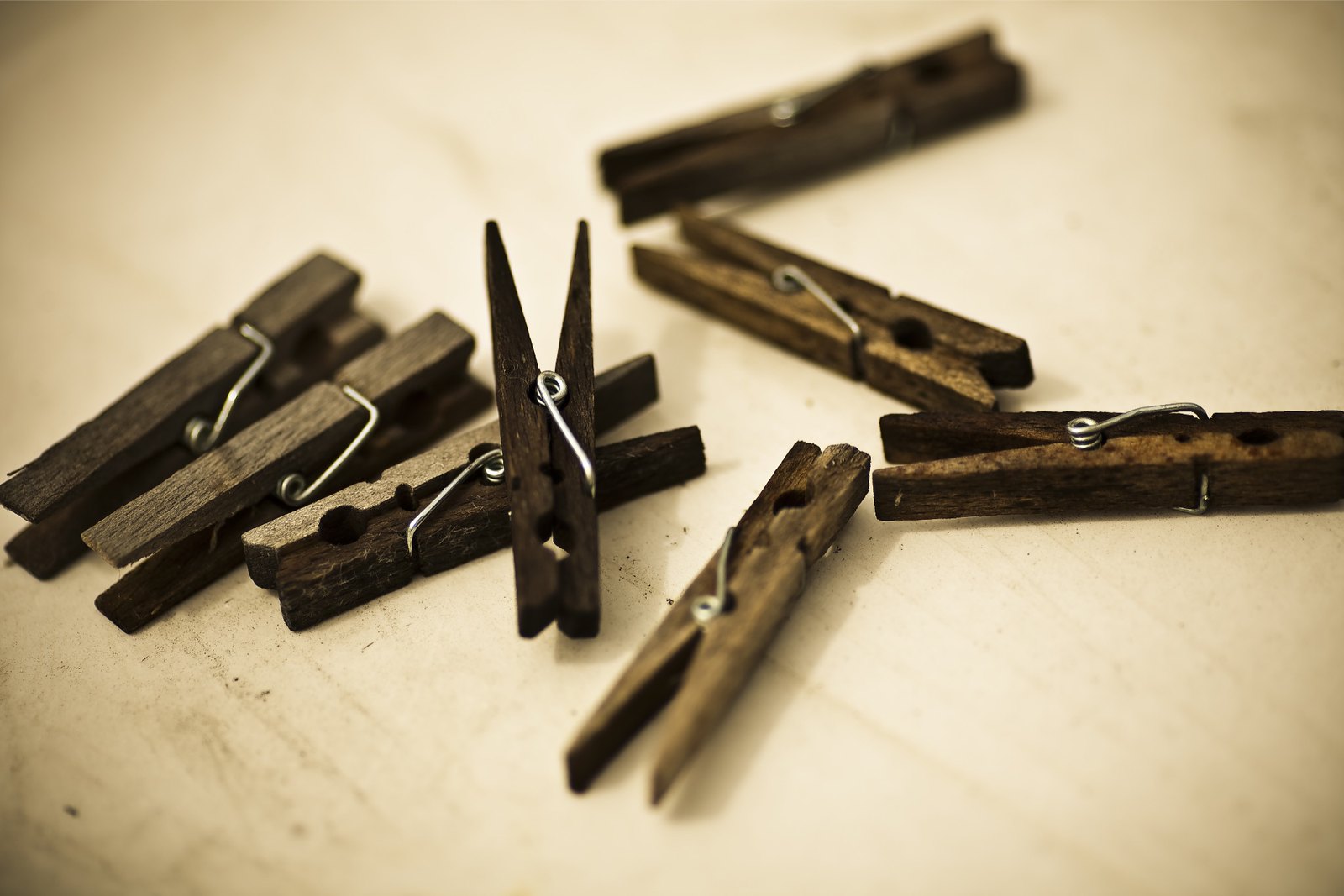This is a close-up, black-and-white photograph showcasing eight heavily weathered wooden clothespins prominently arranged across what appears to be a blonde wooden surface. These clothespins, darkened with age, exhibit various degrees of wear, with some almost entirely black and others showing a bit more natural wood coloration, perhaps due to exposure to elements like rain. The central feature of each clothespin is a sturdy metal spring, seemingly free of rust despite the overall vintage and heavily used look of the pins. Positioned in a somewhat scattered arrangement, the pins on the left side of the image are more clustered, with five visible, while the right side displays the remaining three. The aged appearance of the wood contrasts with the relatively well-preserved metal springs, suggesting that despite their old and worn look, these clothespins remain functional.